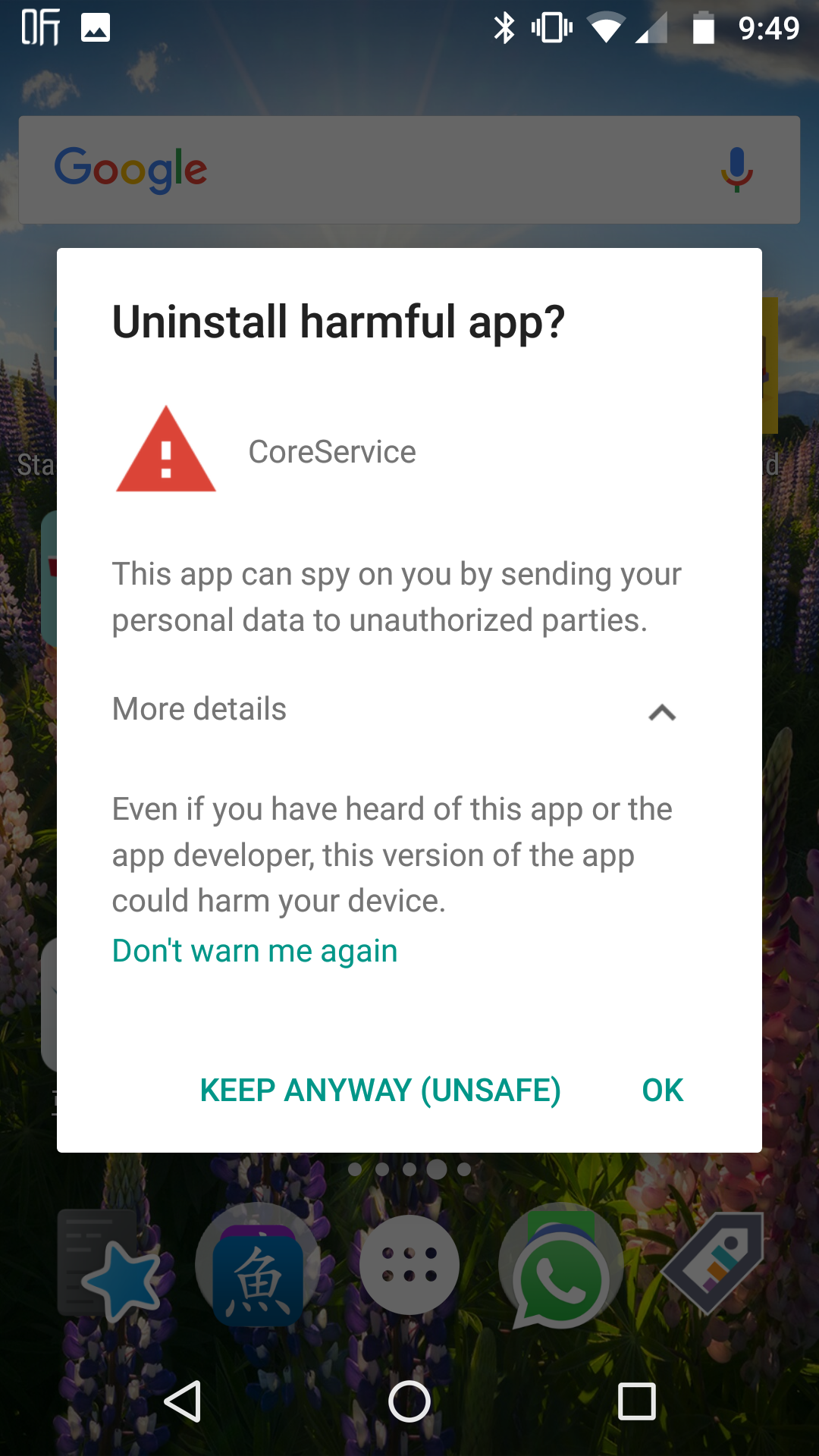A user on an Android phone encounters a pop-up message while viewing their home screen. The pop-up urgently warns: "Uninstall harmful app? Core service. This app can spy on you by sending your personal data to unauthorized parties. More details." The message goes on to state that even if the user is familiar with the app, this version could harm their device. Options provided include "Don't warn me again" and "Keep anyway," the latter marked as unsafe. The home screen, dimmed beneath the pop-up, displays assorted app icons, including one with an Asian character, several messenger apps, and a search bar at the top. The warning message itself has a clean, white background, with links highlighted in a teal color.